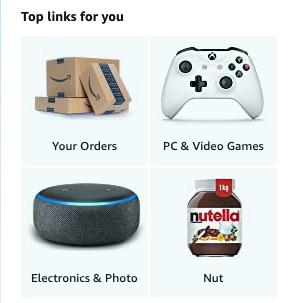A cropped screenshot from an Amazon webpage highlighting four key areas: "Your Orders," "PC & Video Games," "Electronics & Photo," and "Net." 

Each section includes a corresponding image:
1. "Your Orders" features three Amazon cardboard boxes of varying sizes. The smallest box is flat and medium-sized, leaning against the larger two boxes.
2. "PC & Video Games" shows a white Xbox One controller prominently displayed.
3. "Electronics & Photo" displays a black Amazon Echo speaker, identifiable by its fuzzy grille and a blue LED ring near the top, resembling a hockey puck in shape.
4. "Net" showcases a jar of Nutella, with its recognizable branding. 

The rest of the webpage content is cropped out, focusing solely on these four areas and their associated images.